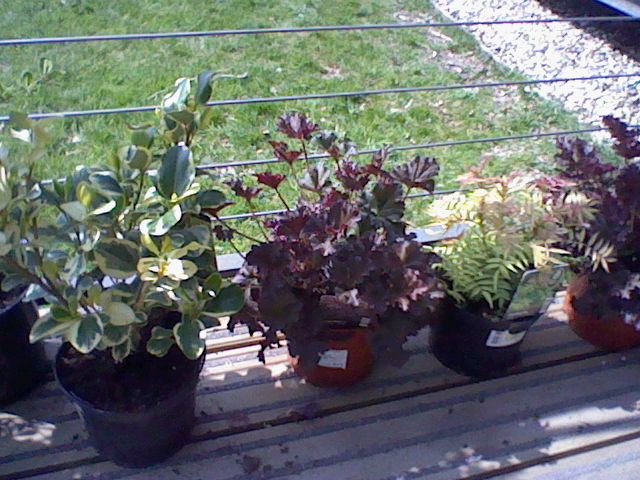This is a low-resolution, blurry photograph of five potted plants arranged on a wooden balcony with a clear view of a yard beyond it. The plants are housed in various planters, with some partially cropped out of the frame. The first plant features green leaves variegated with light yellow and is in a black pot. The second plant resembles a geranium with dark purple to dark red leaves, placed in a terracotta-colored pot. The third plant stands in another black pot, showcasing pale green, narrow leaves ending in points. The fourth pot, similar to the second one, contains another geranium with dark-hued leaves in a terracotta pot. The balcony's flooring consists of decking strips, possibly made of a material like plex, and is bordered by horizontally stretched cable railings. Beyond the deck, the sunny yard displays a green lawn bordered by a white rock bed with patchy grass areas. The angle and cropping of the image accentuate its poor quality, further emphasizing the blurred details.